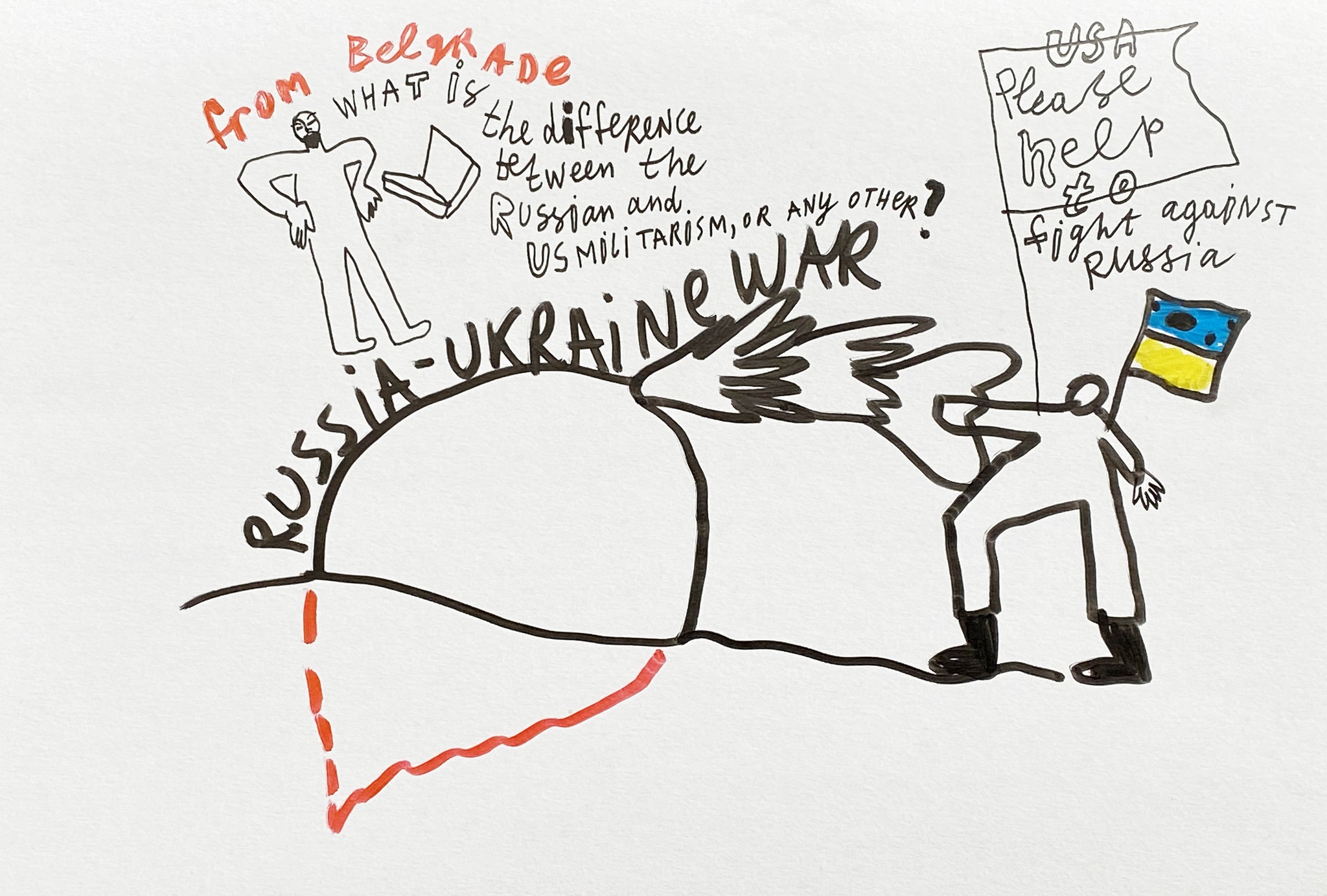This image is a detailed, hand-drawn sketch using various colors and markers on white paper, conveying a multifaceted statement on the Russia-Ukraine war. Central to the image, in black handwriting, is the question: "What is the difference between Russian and U.S. militarism or any other?" Above this text, the orange words "From Belgrade" stand out. Below, in a mix of colors, the phrase "Russia-Ukraine War" is prominently displayed.

To the left of this text, a stick figure with a beard, representing a character from Belgrade, questions the nature of militarism. This figure holds onto what looks like an open laptop, symbolizing communication or possibly the spread of information. Below this figure is a sketch resembling a bomb or a roughly drawn fruit plunging into the ground, with lines extending downward, akin to the roots of a carrot, symbolizing the deep impact and ongoing nature of the conflict.

On the right, another stick figure in combat gear with black boots holds a blue and yellow flag, symbolizing Ukraine. This figure is accompanied by the text on a flag, "USA please help to fight against Russia," written in red. The interplay of these elements suggests a call for international aid and highlights the destructive impacts of the war, visually depicted with vivid use of blue, yellow, black, red, and orange colors.